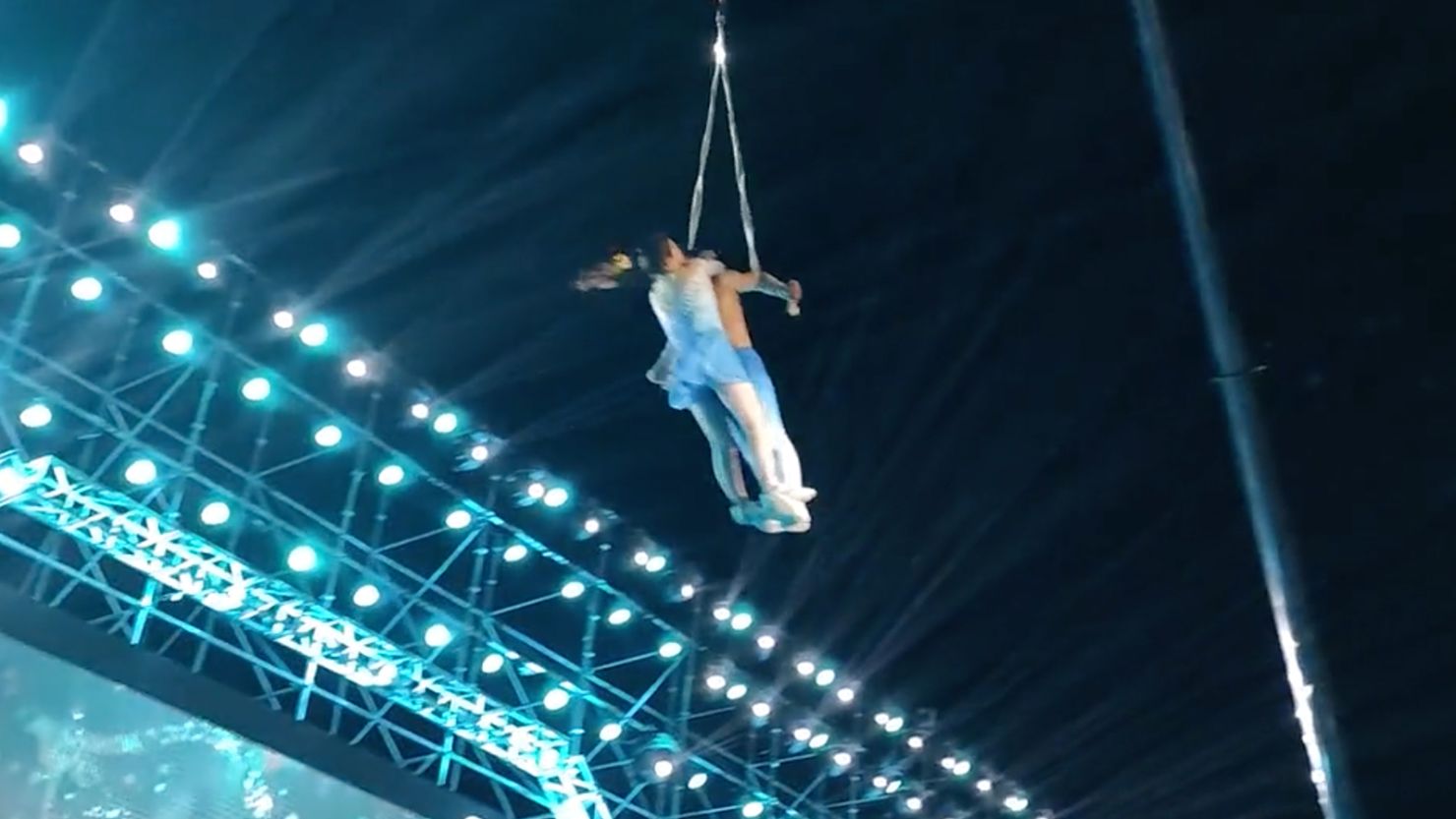This striking photograph captures two acrobats, a man and a woman, executing an aerial stunt high above what appears to be a stadium or a large circus tent. The image is taken from below, offering a dramatic perspective of their daring performance. The acrobats are suspended by silver cables; the man, shirtless and wearing blue shorts, grips these cables tightly while supporting the woman, who clutches him around his chest. She is attired in a light blue skirt and blue athletic shorts, with her hair swept back into a ponytail that flares outward as they spin. 

To the left, towering stadium lights extend from top to bottom, casting a vibrant teal hue that floods the scene. A large screen TV can be seen in the background, enhancing the spectator's view of the performance. The right-hand corner of the image is enveloped in darkness, accentuating the silhouettes of the performers and the silver pole that appears to support the apparatus. The whole setup suggests a grand event with a crowd below, their eyes fixed upward in awe of the acrobats' skill and grace suspended in midair.